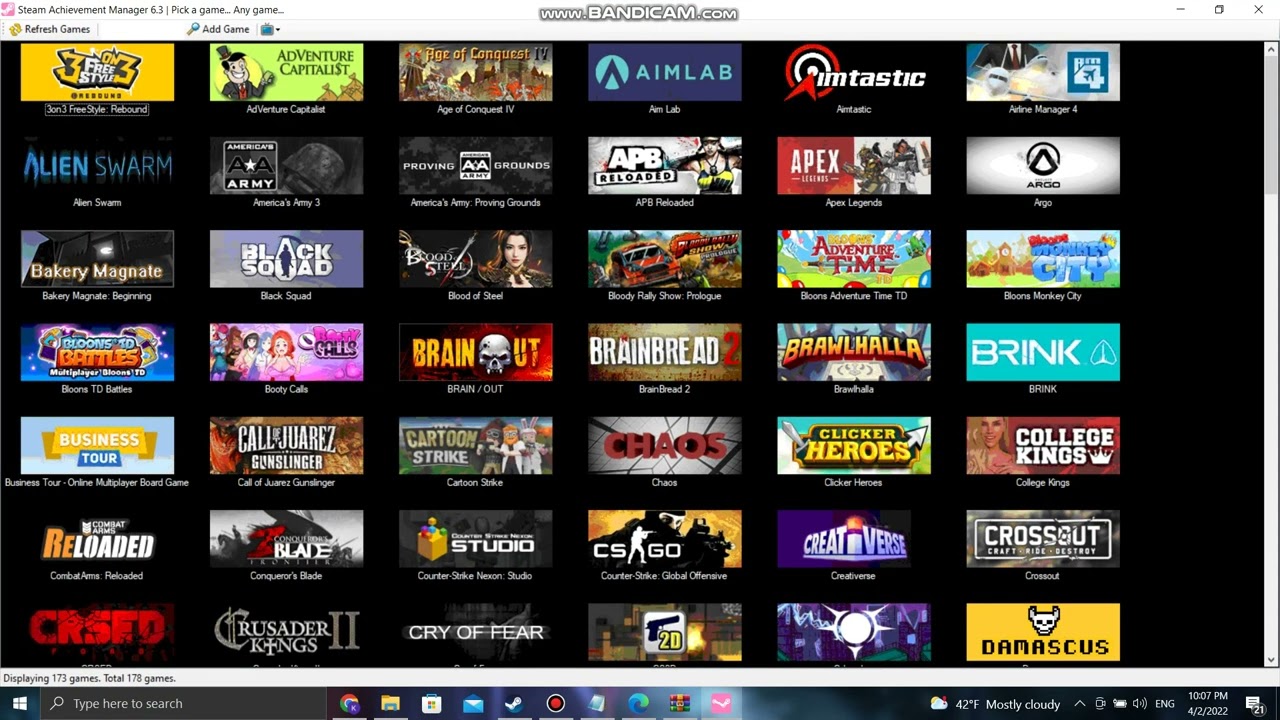The screenshot displays a desktop computer screen featuring a watermark at the top from www.bandicam.com. In the top left corner, there's an open window of "Steam Achievement Manager 6.3," which allows users to manage achievements across games. Within this window, the options to "Refresh Games" and "Add Game" are visible. 

The primary section showcases a large black background with a grid of games listed in alphabetical order. There are seven rows, each containing six games. From left to right and top to bottom, the games are:

1. 3-on-3 Freestyle Rebound
2. Adventure Capitalist
3. Age of Conquest 4
4. Aim Lab
5. Aimtastic
6. Airline Manager 4
7. Alien Swarm
8. America's Army 3
9. America's Army Proving Grounds
10. APB Reloaded
11. Apex Legends
12. Argo
13. Bakery Magnet Beginning
14. Black Squad
15. Blood of Steel
16. Bloody Rally Show Prologue
17. Bloons Adventure Time TD
18. Bloons Monkey City
19. Bloons TD Battles
20. Booty Calls
21. Brain Out
22. Brain Bread 2
23. Brawlhalla
24. Brink
25. Business Tour Online Multiplayer Board Game
26. Call of Warriors Gunslinger
27. Cartoon Strike
28. Chaos
29. Clicker Heroes
30. College Kings